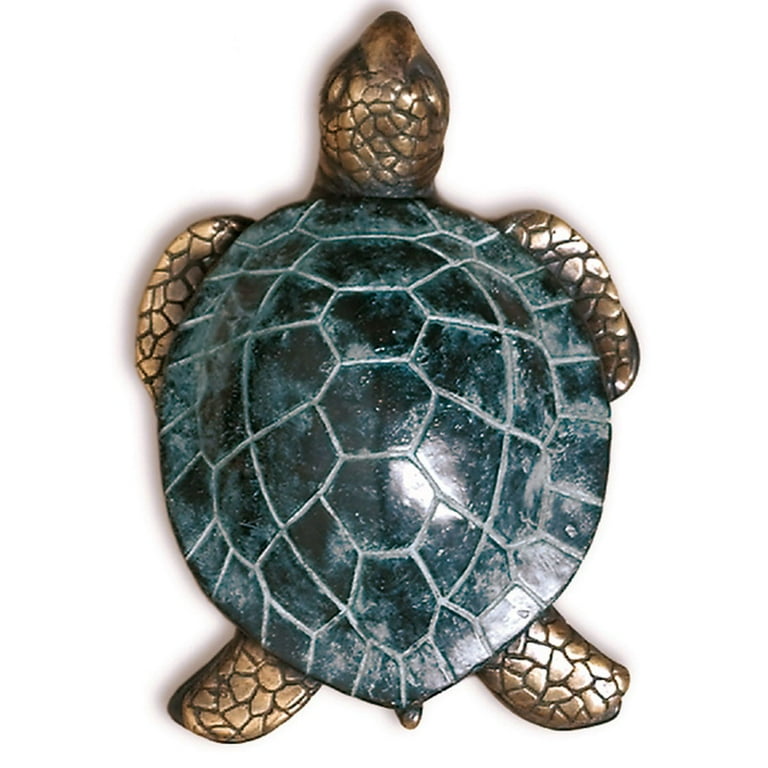The photograph captures an intricately designed turtle brooch or pin, viewed from above. The turtle’s head and limbs are crafted from a gold, brass, or bronze material, intricately detailed to resemble lifelike scales and leather-like skin. The eyes point forward, adding a touch of realism to the piece. The shell is adorned with a hexagonal pattern reminiscent of a natural turtle shell, rendered in a bluish-teal stone—possibly soapstone or marble—with white splotches along the edges. The craftsmanship beautifully combines the metallic and stony elements, creating a striking and elegant piece of jewelry against a white background.